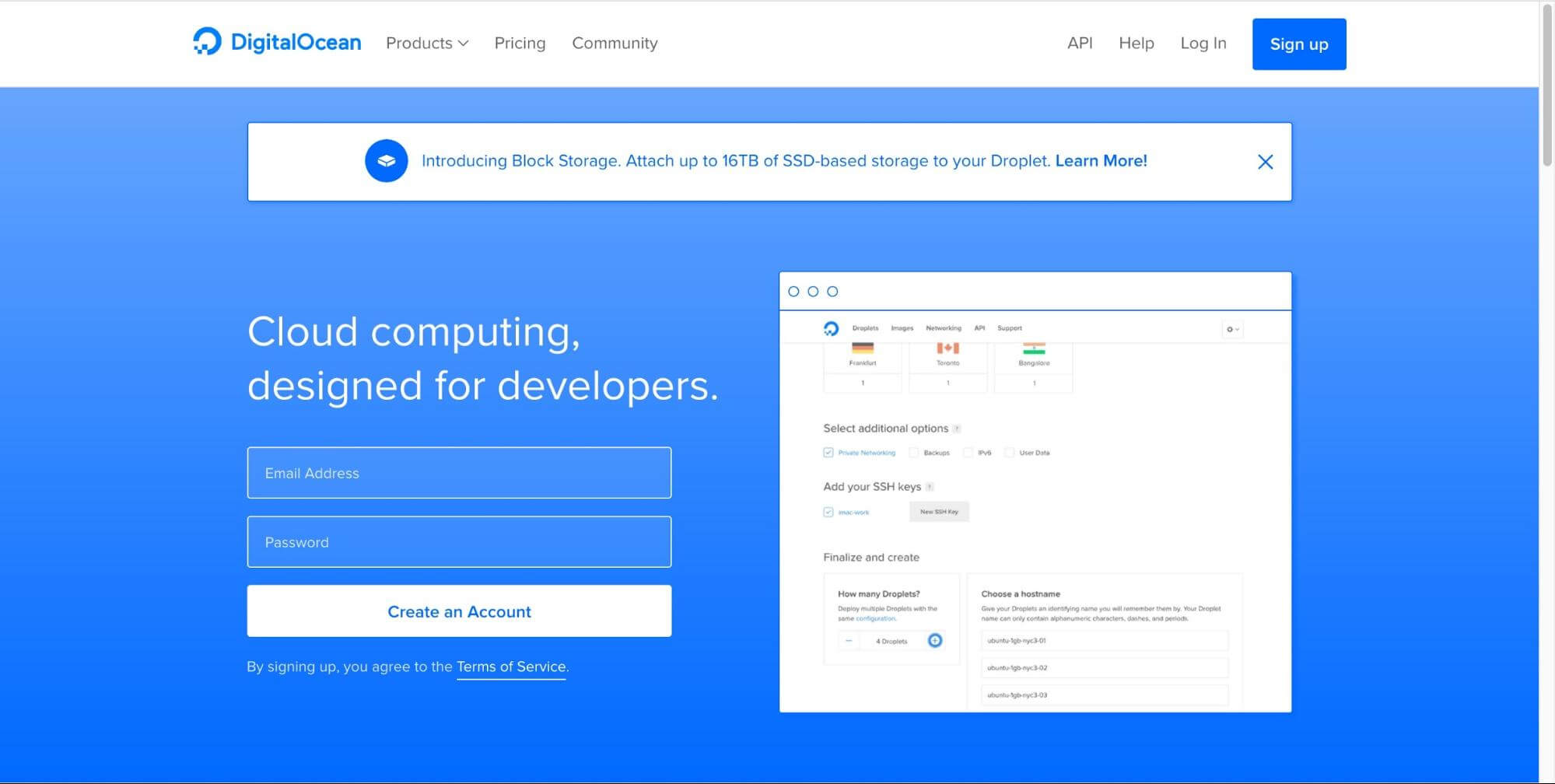The image showcases a webpage from Digital Ocean with a clean, professional layout dominated by a royal blue color scheme. At the top of the page, "Digital Ocean" is prominently displayed in blue text, alongside navigational links for Products, Pricing, Community, API, Help, and Login. 

The center of the screen features a white opt-in form where users are prompted to sign up, with a highlighted blue "Sign Up" button catching the eye. Above this form, there's an informational prompt introducing "Block Storage," noting that users can attach up to 16TB SSD-based storage. This text is also in blue.

Further down, the form invites users to enter their email address to create an account. Hidden in the lower section, there's a barely visible button that allows users to edit their information, enhancing ease of use for developers interested in cloud computing solutions.